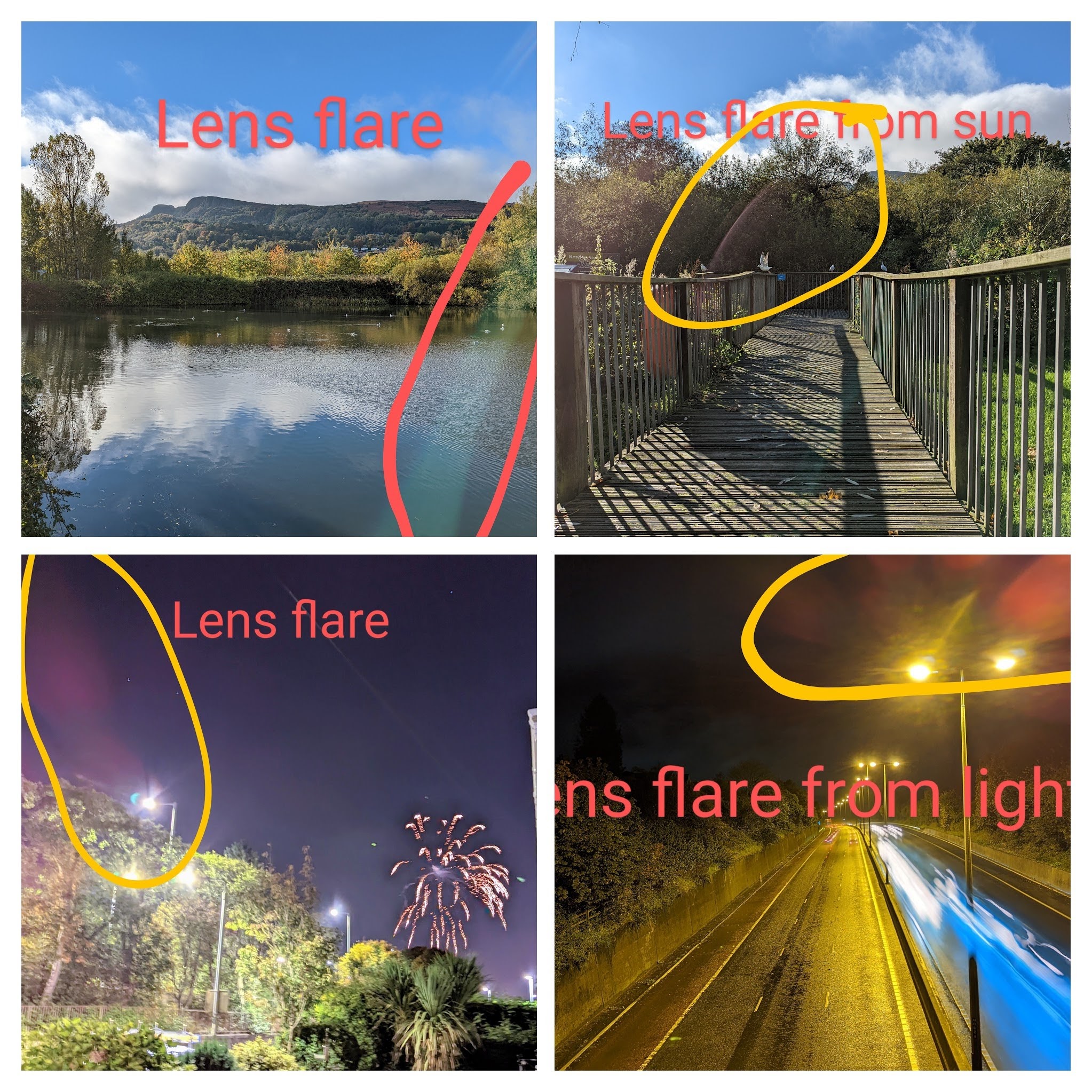This image collage comprises four distinct landscapes, each highlighting a lens flare with hand-drawn circles and captions. The top-left photo captures a serene body of water bordered by trees, bushes, and mountains, under a clear blue sky dotted with clouds. A red circle denotes the lens flare, labeled "lens flare." The top-right photo showcases a wooden walkway bridge amidst a verdant setting of trees and grass, with a yellow circle around the lens flare and the caption "lens flare from Sun." The bottom-left image features a nighttime scene with various green and palm trees, street light poles, and a firework illuminating the sky; here, a yellow circle marks the lens flare labeled "lens flare." Lastly, the bottom-right picture depicts an empty highway at night, flanked by light poles and trees, with a yellow circle around the lens flare, captioned "lens flare from light."